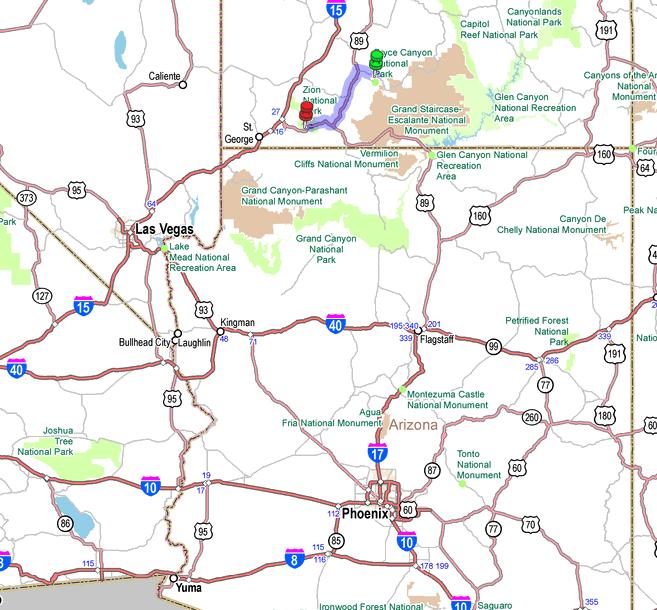This detailed map prominently features the state of Arizona and highlights various key locations. The cities marked on the map include Bullhead City, Laughlin, Kingman, and Flagstaff, along with the significant landmark, Petrified Forest National Park. Major highways are indicated, including Interstate 15, Interstate 10, Interstate 40, and Interstate 17, as well as Highway 191. The map's design utilizes red lines to delineate roads and highways, while blue indicates bodies of water. Additional notable sites featured on the map are Canyonlands National Park, Capitol Reef National Park, Zion National Park, Tonto National Monument, and Ironwood Forest National Monument.